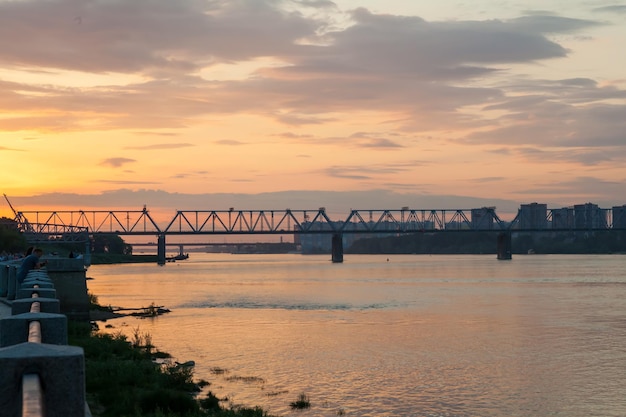The photograph captures a serene river scene at sunrise or sunset, with a calm expanse of water that shows no signs of boat activity. Dominating the middle of the image is a bridge spanning the river, supported by three prominent columns. The bridge's structure includes both a trestle for trains and support rails overhead, piecing it into about four visible sections. The water underneath is mostly smooth with only slight ripples, framed by low-lying marine plants along the edges. To the right, the city skyline suggests an industrial district, marked by buildings and construction equipment, though no human activity is apparent on the bridge or the water itself. The sky takes up the top half of the image, painted in warm hues of yellow, orange, red, and light blue, indicative of either a sunrise or sunset. Adjacent to the water on the bottom left is a railing in blue and brown tones, and a few people can be spotted along this riverside walkway, adding a subtle touch of life to the scene.